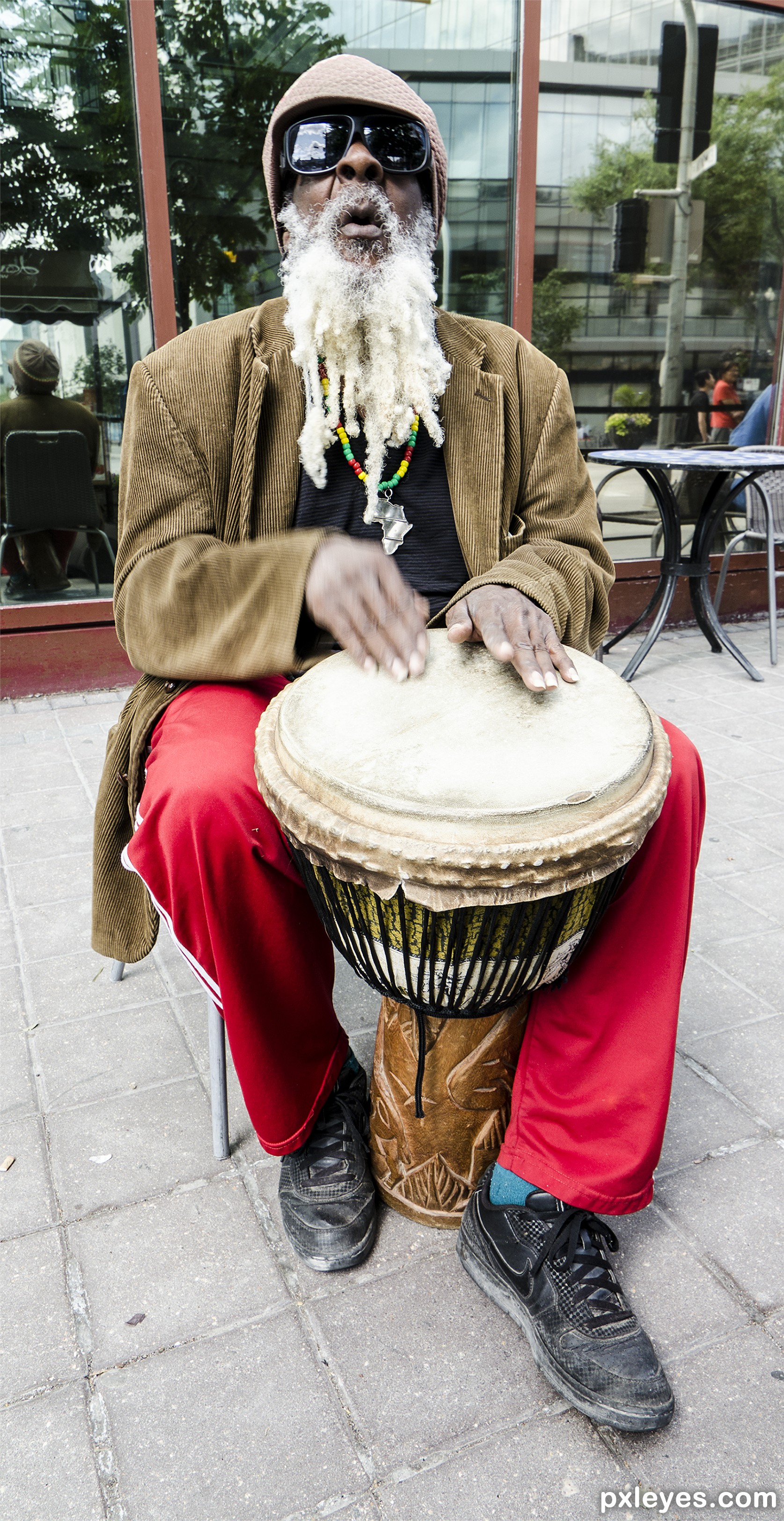In this detailed photograph, an elderly black man, possibly blind, is deeply immersed in playing a large bongo drum nestled between his legs. He sits on a chair positioned on a sidewalk in front of a café-style building with glass window panes, reflecting both the street across and his own image. His attire is eclectic and vibrant: he dons black sneakers, a single blue sock, bright red pants, a long brown corduroy coat, and a black t-shirt. Around his neck hangs an African continent-shaped necklace adorned with red, yellow, and green beads, infusing his outfit with a touch of vibrant culture. His distinctive long white beard, styled in dreadlocks, complements his dark skin, and his eyes are concealed behind large, oversized black sunglasses. Topping off his look is a tan cap. The drum, with its narrow base and wider cream-colored top where his skilled hands play rhythmically, adds to the musical ambiance. A small black table is visible directly behind him, adding to the café atmosphere, which further highlights the serene yet lively street setting he is part of.